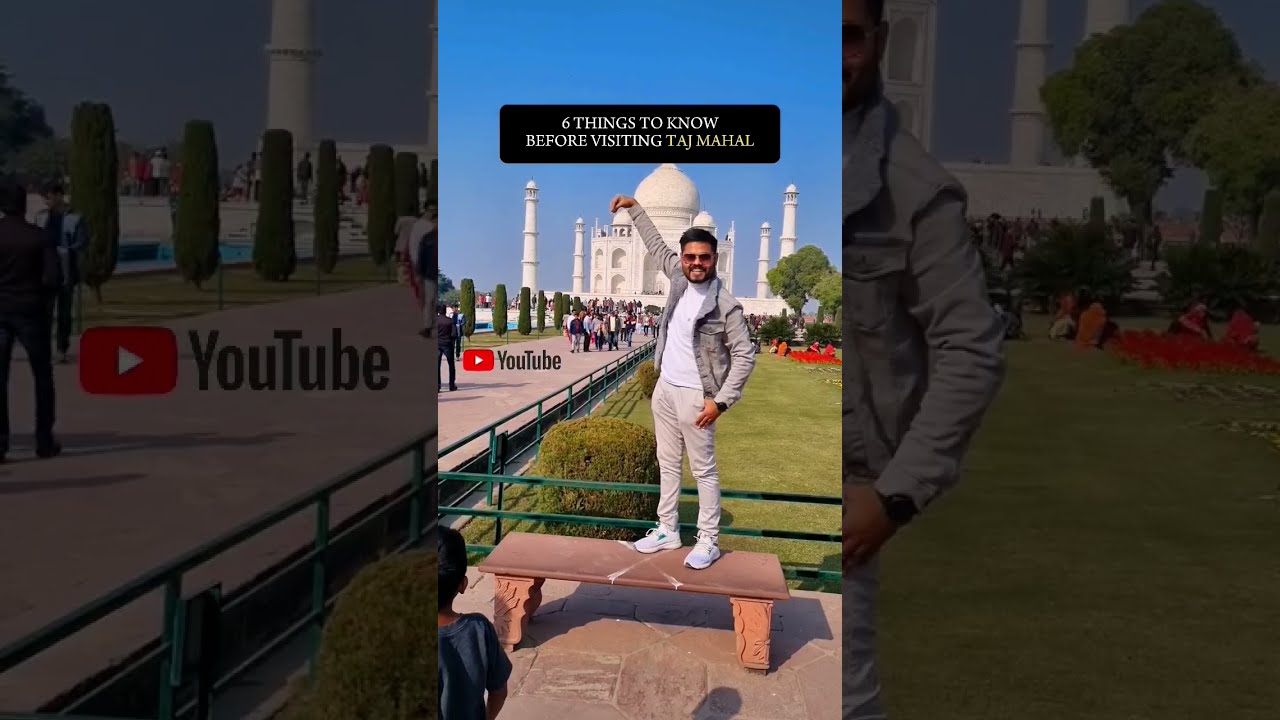In this detailed image, a YouTube screenshot focuses on a man posing creatively in front of the Taj Mahal. The central figure, a brown-skinned man with thick black hair that stands three to four inches tall, is standing on a rust-colored marble bench with a concrete base, situated atop rust-colored tiles. He is wearing a gray jacket over a white shirt, white pants, white shoes, and black sunglasses. 

The man is playfully using perspective to make it appear as if he is interacting with the Taj Mahal behind him. His right arm is raised and curved, seemingly cupping one of the smaller domes of the Taj Mahal due to the camera angle. His left hand is in his pocket with his fingers pointing down.

The backdrop features the majestic, all-white Taj Mahal, clearly identifiable despite a subtle black color filter over the entire scene. The architectural wonder is complemented by a central large dome and smaller domes flanked by six thin pillars, three on each side. A green metal fence guides visitors toward the building, and the surrounding landscape includes a well-maintained garden of tall shrubs, trees, and a lush lawn.

Numerous people can be seen walking along the garden path and a noticeable red carpet area. The image is sunny, adding to the vibrant ambiance. The top center of the image contains white text on a black background that reads, "Six Things to Know Before Visiting the Taj Mahal," highlighting the content of the YouTube video. The iconic YouTube logo is also visible in the image, confirming its origin from the platform.